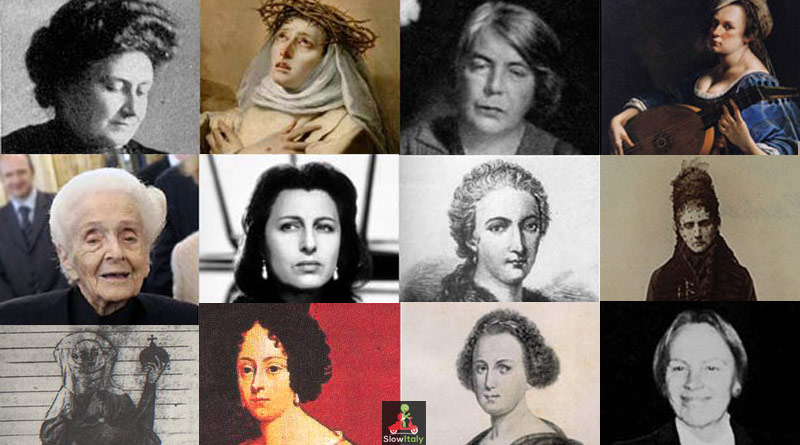The image is a detailed collage consisting of 12 photos of women, arranged into three rows and four columns, showcasing various stages and aspects of their lives. Predominantly featuring women from different eras, most seemingly from the 1700s or 1800s based on their clothing and hairstyles, the photos alternate between black and white and colored images. In the top row, the first and third images are black and white, with the first depicting a woman in traditional attire. The second image is in color and shows a woman wearing a crown of thorns, while the fourth image has a woman in a blue dress playing a stringed instrument, also in color. Each row below mirrors the layout with a mix of black and white and colored photos, presenting a tapestry of both older and younger women. The bottom-left photo is black and white, followed by a colored image, another black and white, and ending with a color photograph. A small red scooter is depicted in the lower portion, with the text "Slow Italy" at the bottom, alluding to a narrative enriched by these high-quality images, collectively suggesting a historical journey through time and personal stories.